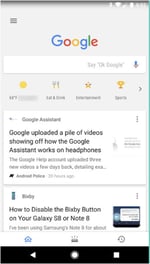A screenshot of a Google search results page appears as a slightly blurry image, possibly captured from an older smartphone. The primary focus is on a news article showcasing a series of videos uploaded by Google, demonstrating the functionality of Google Assistant when used with headphones. Beneath this article, another headline explains how to disable the Bixby button on Samsung Galaxy devices. The overall quality of the image suggests it may have been taken some time ago, emphasizing the now-outdated technology of the phone used to capture this screenshot.